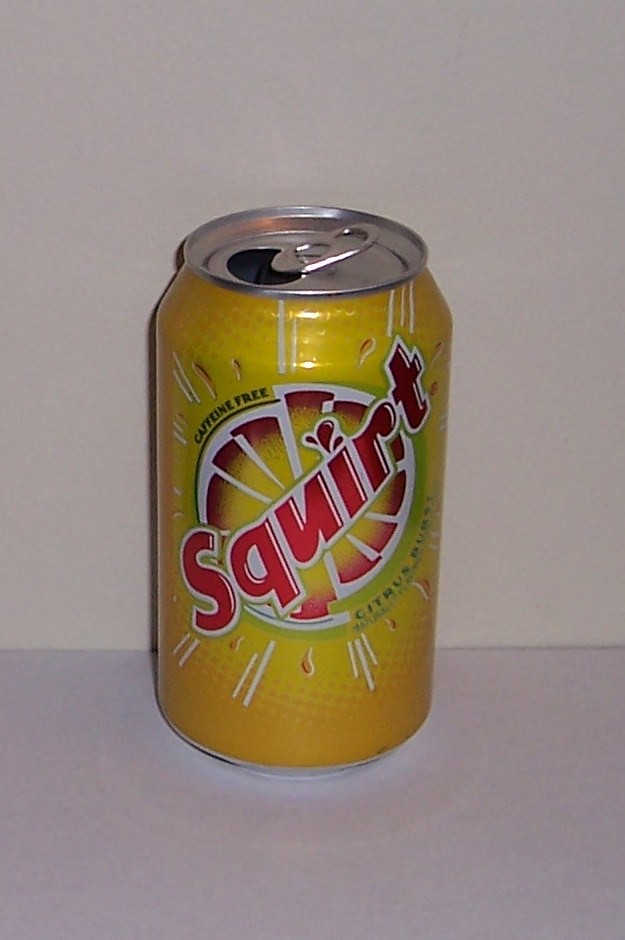This is a vibrant photograph capturing a can of Squirt soda set against a purplish-gray countertop with a white painted wall as the backdrop. The can features a shiny, metallic finish with an eye-catching orange and yellow design. At the center of the can is the bold Squirt logo, written in large red letters with distinctive highlighting. Just beneath the branding, there is a cartoonish depiction of a sliced citrus fruit—perhaps an orange, grapefruit, or even a lemon—rendered in shades of red, yellow, and orange. The can has been opened, adding a touch of realism to this detailed and visually appealing composition.